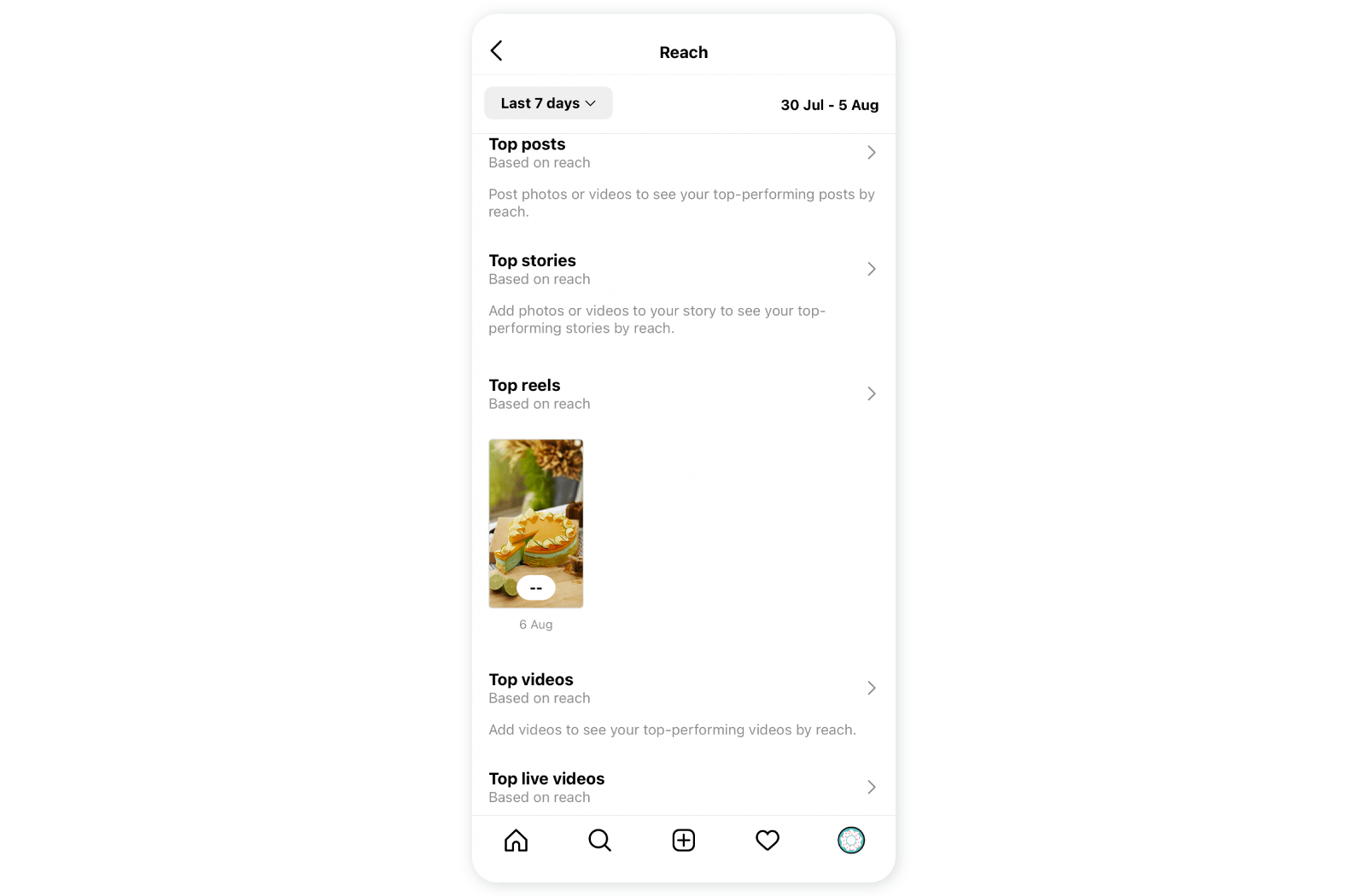The image depicts a page on a mobile phone, likely from a social media platform, with a clean white background and black text. At the top, the word "REACH" is prominently displayed, followed by the text "Last 7 days," with the date range specified as 30th of July to the 5th of August. This section appears to be an analytics overview for the user's posts.

Beneath this heading, there are two subsequent sections. The first is titled "Top posts based on REACH," which encourages users to post photos or videos to identify their top-performing content based on reach. The second section is titled "Top stories based on search," suggesting that users add photos or videos to their stories to see their best-performing content in that category.

As part of the visual content, the page features an image of a cake with a caramel topping. A slice has been cut and pulled away, revealing a light aqua-colored cream inside that might be pistachio-flavored. The cream sits atop visible sponge layers.

Further down, the page lists categories such as "Top videos" and "Top live videos." At the very bottom of the screen, there is a navigation bar with icons for Home, Search (a magnifying glass), Notifications (a heart), Settings, and an option to Add content (a plus sign inside a square). The layout is straightforward, with a focus on user engagement and content performance.